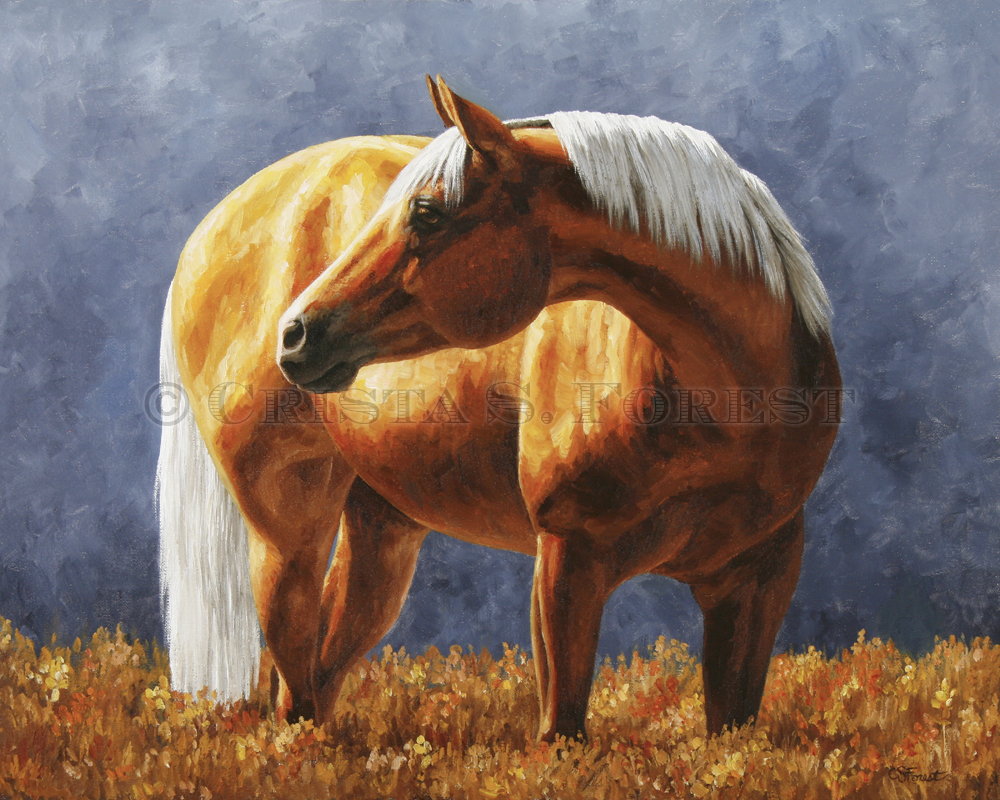The artwork is a digital painting featuring a chestnut brown horse with tan highlights standing in a golden wheat field. The horse has a distinctive white mane, a tail that cascades down to the ground, and a white patch on its forehead. It is posed with its head slightly turned back, offering a side view of its elegant profile. The background is a serene blue sky, as if the horse is on a hill with nothing but open sky behind it. The field of yellow and white vegetation beneath the horse adds a rich textural element to the scene. The signature "Christa S. Forest" is lightly visible across the painting. The overall color palette includes shades of brown, white, and blue, contributing to the artwork's tranquil and natural ambiance.